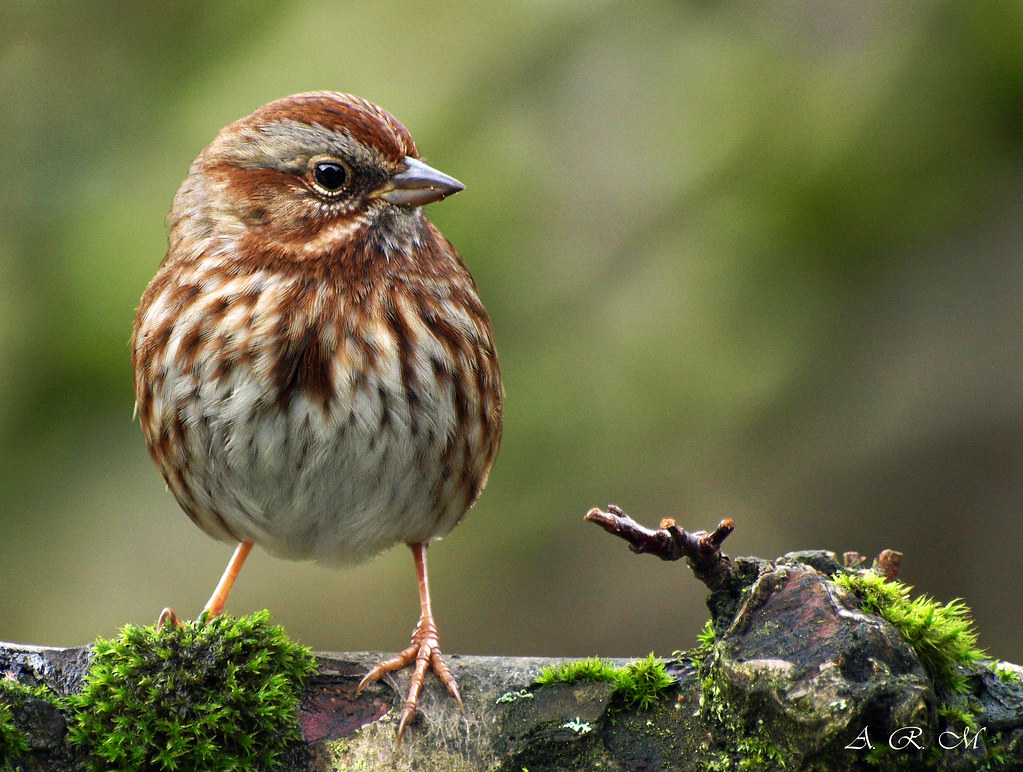The image captures a close-up of a tiny songbird perched on a moss-covered branch against a backdrop of muted greens and beiges, suggesting a forest setting. The bird has a small body with brownish-red legs and webbed feet. Its plumage features a white belly with brown streaks, while its wings and back display a striped pattern of browns and grays, imparting a textured appearance. The head of the bird is adorned with alternating stripes of reddish brown and gray, emphasizing its detailed feather patterns. The bird's small gray beak and clear black beady eye are prominently visible as it looks off to the right. The bottom right corner of the image contains the photographer's cursive initials, A-R-M.